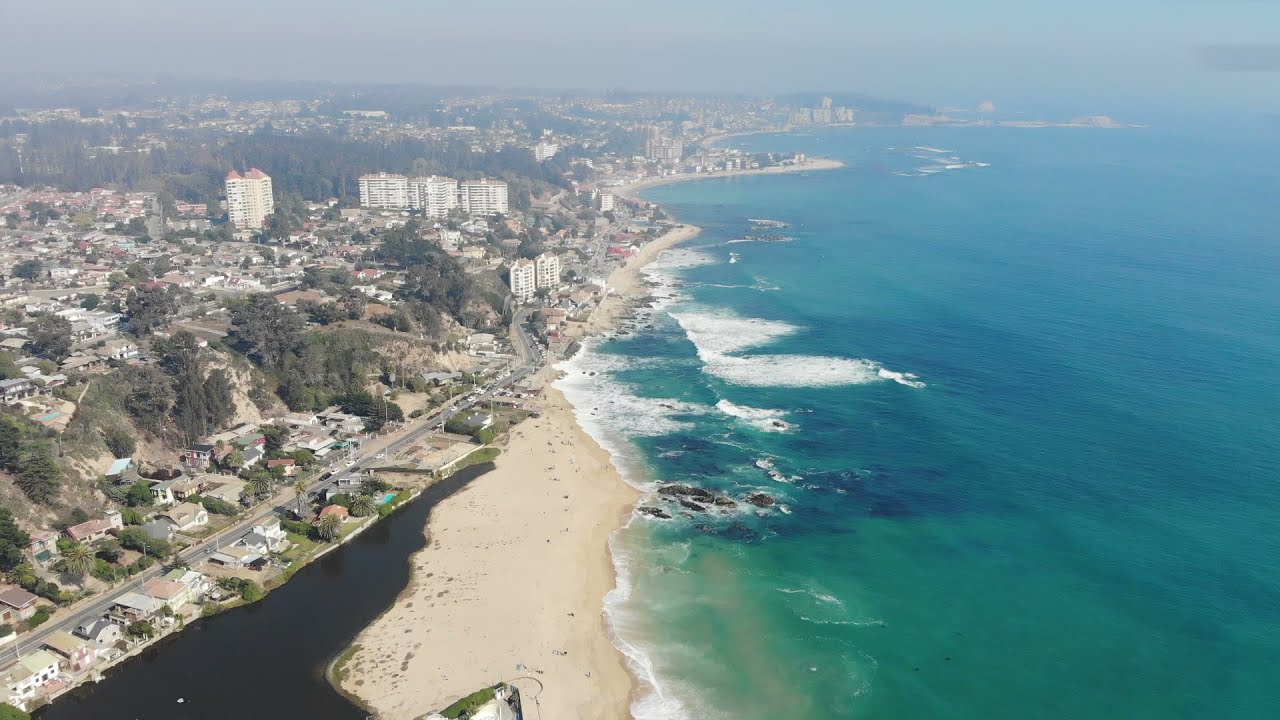This detailed aerial photograph captures an expansive view of a coastal town on an overcast day. To the right of the image, the deep blue and aqua ocean stretches into the horizon, with white waves breaking against a bright sandy beach that curves away into the distance. Central to the photograph, the beach is bordered by rocks and shoals that add texture to the shoreline. On the left side of the image, a coastal highway winds its way from the bottom left corner into the distance, lined with low houses with dark roofs and several high-rise, predominantly white structures such as hotels, apartments, and commercial buildings. These tall buildings stand prominently amongst a dense array of trees and additional buildings that fade into the misty, smoggy background, making the far distance almost indiscernible. The urban landscape, marked by the presence of numerous buildings along the cliffs and shoreline, suggests a bustling tourist destination, though the streets and beach appear relatively devoid of people at this moment. The overall effect is a realistic and detailed snapshot of a coastal community seamlessly blending into the natural beauty of the ocean and beach.